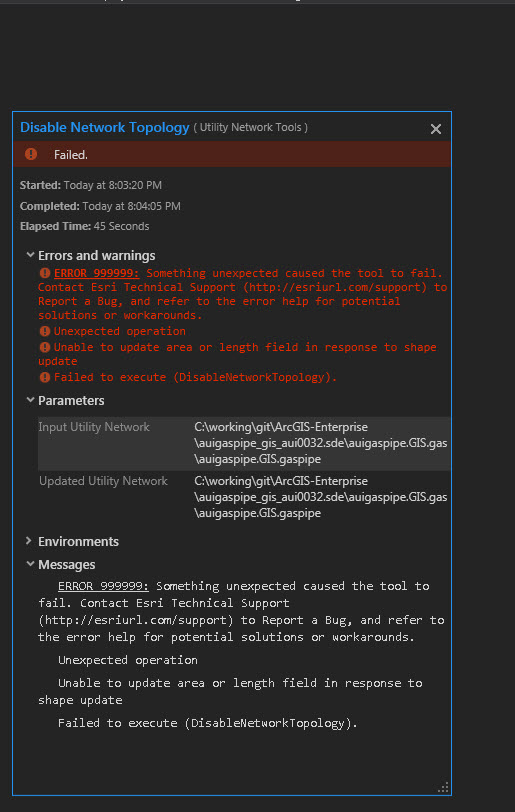The image displays a user interface with a black background, prominently featuring text and icons associated with a network operation. At the top, enclosed in a blue box, the text reads "Disable Network Topology," with "Utility Network Tools" in gray parentheses beneath it. Directly below this, a red box contains a red circle with an exclamation mark in the center, along with the word "Failed" in bold white text. Underneath, a gray subtitle states, "Started today at 8:03:20 PM, completed today at 8:04:05 PM," followed by "Elapsed time: 45 seconds."

Further down, an arrow points downward to a section labeled "Errors and Warning" in white text. This section contains another red circle with an exclamation mark, and accompanying red text that reads, "Error 999999: Something unexpected caused the tool to fail. Contact technical support." It also mentions a URL for reporting a bug and suggests referring to the error help for potential solutions or workarounds. The final line of text, in gray, states, "Unexpected operation."